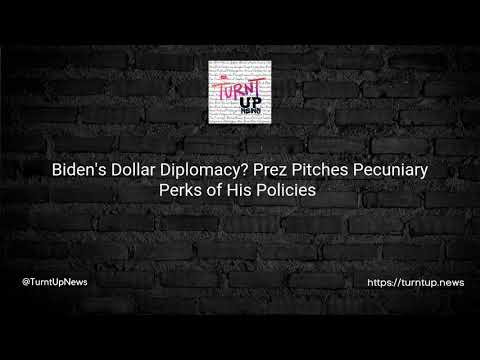The image showcases an ad set against a black brick wall backdrop with lighter mortar lines outlining the bricks. Centrally located at the top is a logo that reads "Turn It Up" in pink and black. Directly beneath the logo, white text boldly declares, "Biden's Dollar Diplomacy? Press pitches pecuniary perks of his policies." To the bottom left corner, the handle "@turnitupnews" is prominently displayed, while the bottom right corner features the URL "https://turnitup.news." The only color elements in the image are the "Turn It Up" logo, making it stand out against the monochromatic brick wall background. The design suggests it could be a digital advertisement or promotional content for a podcast or news segment.